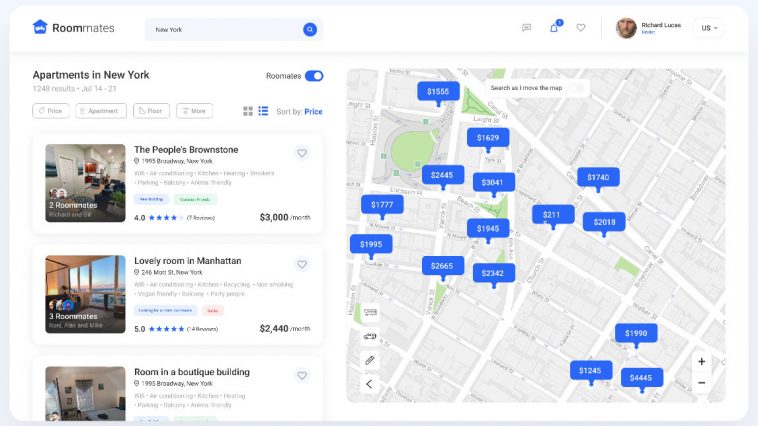Here is a cleaned-up and detailed caption for the image described:

---

The image depicts the landing page of a website called "Roommates," presented in a landscape rectangular format, approximately twice as wide as it is high. The page features a white background with a light bluish-gray border, thicker on the sides compared to the top and bottom. At the top left corner of the header, there's a blue house icon with an indented white shape, next to the bolded word "Roommates"—the "Room" part in a darker shade than "mates." To its right, a long rectangular search bar with a light blue background displays the words "New York" in gray, accompanied by a blue search icon with a white magnifying glass in the center.

Towards the upper right corner, a dropdown box labeled "U.S." allows country selection. Beside it, a user avatar of a bearded man with Caucasian skin and reddish hair appears, labeled "Richard Lucas" in bold text with an additional unidentifiable label below. A thin vertical gray bar separates this section from three icons: a heart outline, a bell with a notification badge, and a flag icon.

Beneath this busy header, a light gray line spans the width. The main content is divided into two sections: a 45% panel on the left featuring words and pictures of apartments, and a 55% section on the right showing an overhead road map.

The map is light gray with white roads, some marked as highways, and green areas representing five parks. Fifteen medium blue rectangles with rounded corners and white price texts act as pin drops, displaying various four-digit apartment prices, except one at $211. In the center, a white search bar reads "search as" followed by unreadable text. Four icons (including a pencil, an arrowhead, and a car) appear in the lower left corner, and a plus-minus zoom control is at the lower right.

The left panel highlights three apartment listings. "The People's Brownstone," priced at $3,000 per month, features a star rating of 4.0 and seven reviews. Below it, "Lovely Room in Manhattan" is priced at $2,440 with a perfect 5.0 star rating. The final listing, "Room in a Boutique Building" on Broadway, New York, is partially visible with a cut-off star rating and price.

---

This cleaned-up caption maintains detailed observations and information provided in a structured manner.